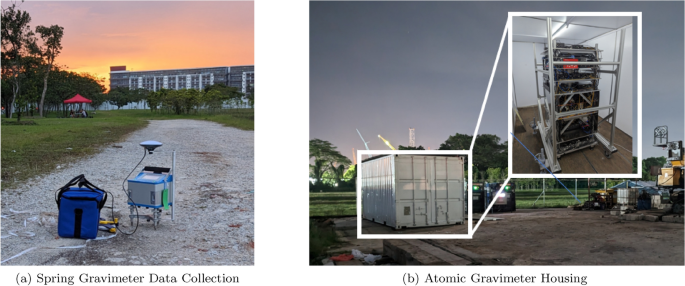The combined image showcases two photographs depicting advanced gravimetric equipment in outdoor settings. On the left, a labeled photograph titled "Spring Gravimeter Data Collection" features a scientific device positioned on a dirt or gravel road. The road leads to a distant multi-story building flanked by trees and grass, with a red awning off to the side providing shade for people beneath it. The sunset sky casts a beautiful glow over the scene. To the right, another labeled photograph, "Atomic Gravimeter Housing," focuses on a steel storage container, potentially transported by a truck. The open container reveals shelves holding various machinery inside. This equipment is set in a yard with additional nearby structures and trees, under a gray, cloudy evening sky transitioning to nighttime.